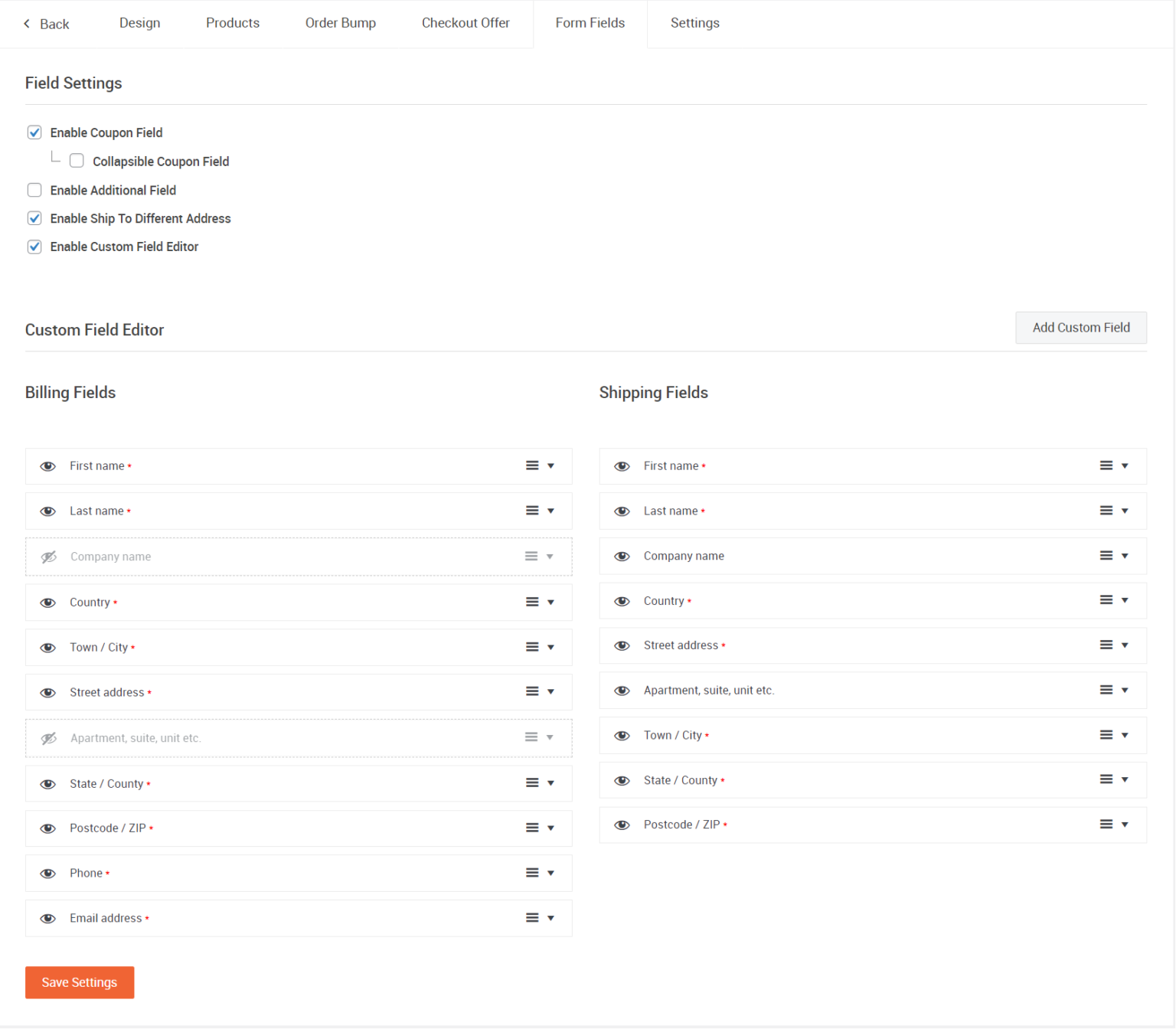Screenshot Description:

The screenshot depicts the "Field Settings" menu interface, showcasing various configurable options for form customization. Below the main title, there is a list of options, each accompanied by a checkbox on the left to enable the feature. The options listed are:

1. **Enable Coupon Field**: Checkbox checked.
2. **Collapsible Coupon Field**: Checkbox checked.
3. **Enable Additional Field**: Checkbox unchecked.
4. **Enable Ship to Different Address**: Checkbox checked.
5. **Enable Custom Field Editor**: Checkbox unchecked.

Further down, the "Custom Field Editor" section is visible, categorized into "Billing Fields" and "Shipping Fields", each expandable through a drop-down arrow on the right.

**Billing Fields** contains approximately 12 categories:
- First Name  
- Last Name  
- Company Name  
- Country  
- Town/City  
- Street Address  
- Apartment/Suite  
- State/County  
- Postcode/Zip  
- Phone  
- Email Address

Each category is complemented by an information icon (i) on its right, presumably providing additional details or tips.

**Shipping Fields** displays a similar structure to the Billing Fields with categories:
- First Name  
- Last Name  
- Company Name  
- Country  
- Street Address  
- Apartment/Suite/Unit, etc.  
- Town/City  
- State/County  
- Postcode/Zip

These fields also feature the information icon (i) for further guidance on each category.